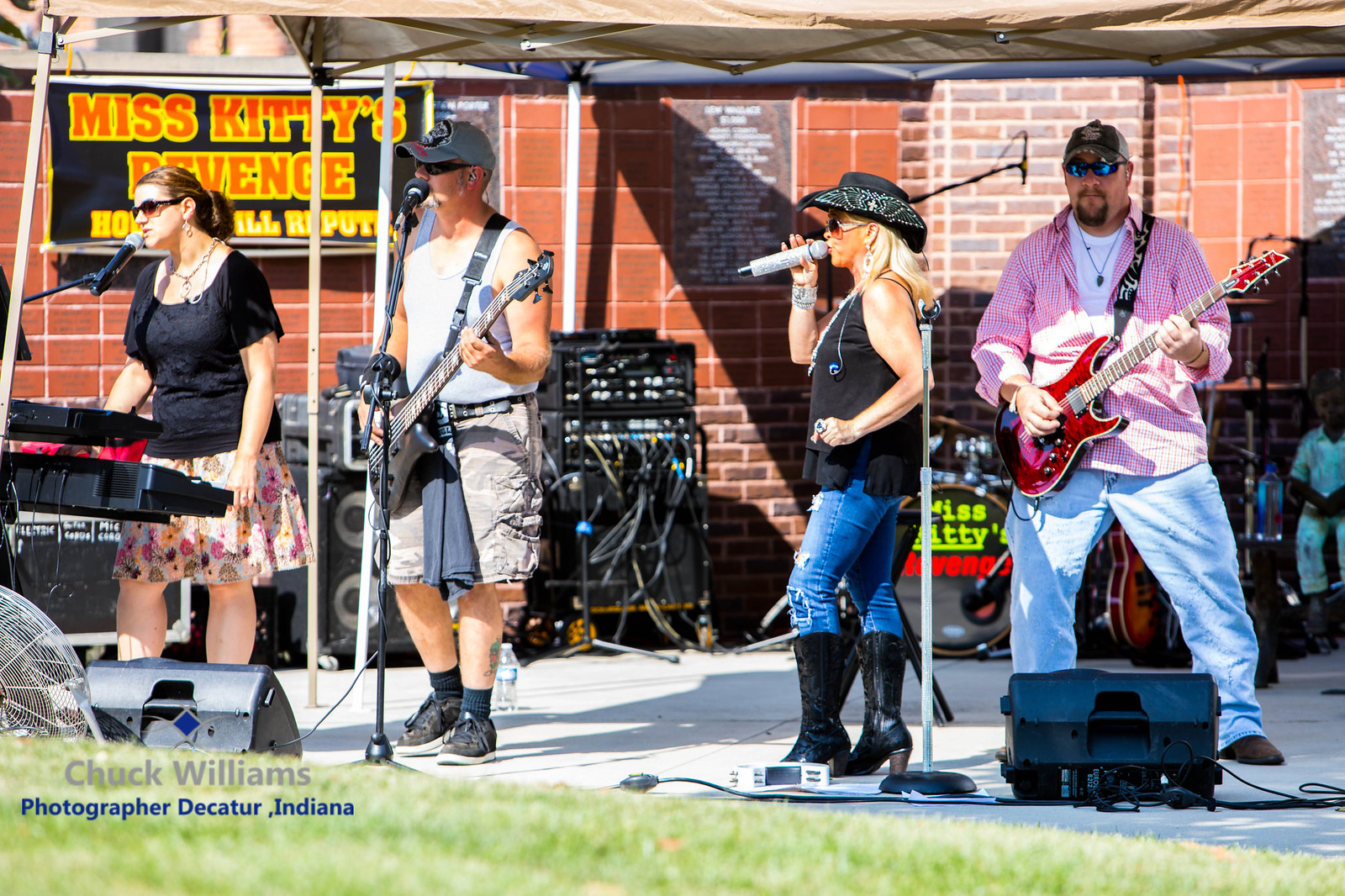This photograph, taken by Chuck Williams in Decatur, Indiana, depicts an outdoor performance by the country-rock band "Miss Kitty's Revenge." The band is positioned on a cement surface beneath a tent, with some grass visible in the foreground and a red brick wall forming the backdrop. A banner and the band's drum set both feature the name "Miss Kitty's Revenge." 

The female lead singer stands out with her blonde hair, black cowboy hat adorned with a cross, blue denim jeans, black cowboy boots, and a sleeveless black top; she is singing into a microphone. To her left, the guitarist is a heavier-set man wearing jeans, a pink and red plaid button-down shirt over a white t-shirt, a ball cap, and fluorescent blue sunglasses; he plays a red guitar and also sings into a microphone. On the far left, the other male guitarist, who sings as well, is dressed in a ball cap, black sleeveless tank top, cargo shorts, and dark shoes. He plays a black bass guitar. The woman on keyboards is dressed in a patterned pink skirt, a short-sleeved black top, and sunglasses, and she, too, sings into a microphone. The group’s speakers are set up on the ground in front of them, completing the scene of this lively outdoor musical event.